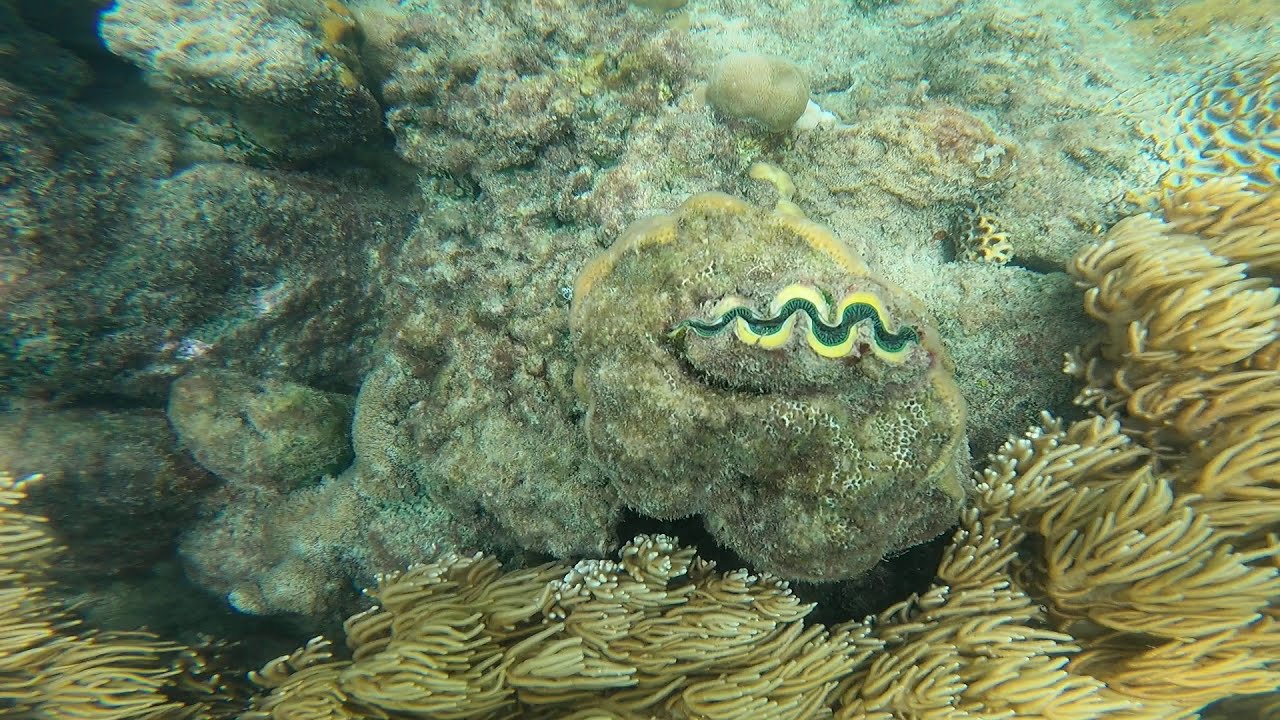This is a highly detailed close-up view of an underwater scene, possibly within a coral reef. The image captures a lush and diverse marine ecosystem. Along the bottom and rising diagonally from the bottom left to the top right, there are dense growths of long, flowing structures resembling seaweed or anemones, which range in color from golden-yellow to taupe. Amongst these, the main focal point emerges as a hand-drawn, serpentine figure that appears almost snake-like or eel-like in shape. This figure, centrally positioned, stands out with its dark green body accented by a light yellow border. Surrounding this focal point is a background filled with shades of light and dark green, which might represent rocky areas or coral formations. Additional textures and colors, including a sandy gray and mossy tones, provide a rich, varied backdrop. The entire scene lacks any signs of human presence or typical fish, focusing instead on the texture and color complexity of the marine life and environment.